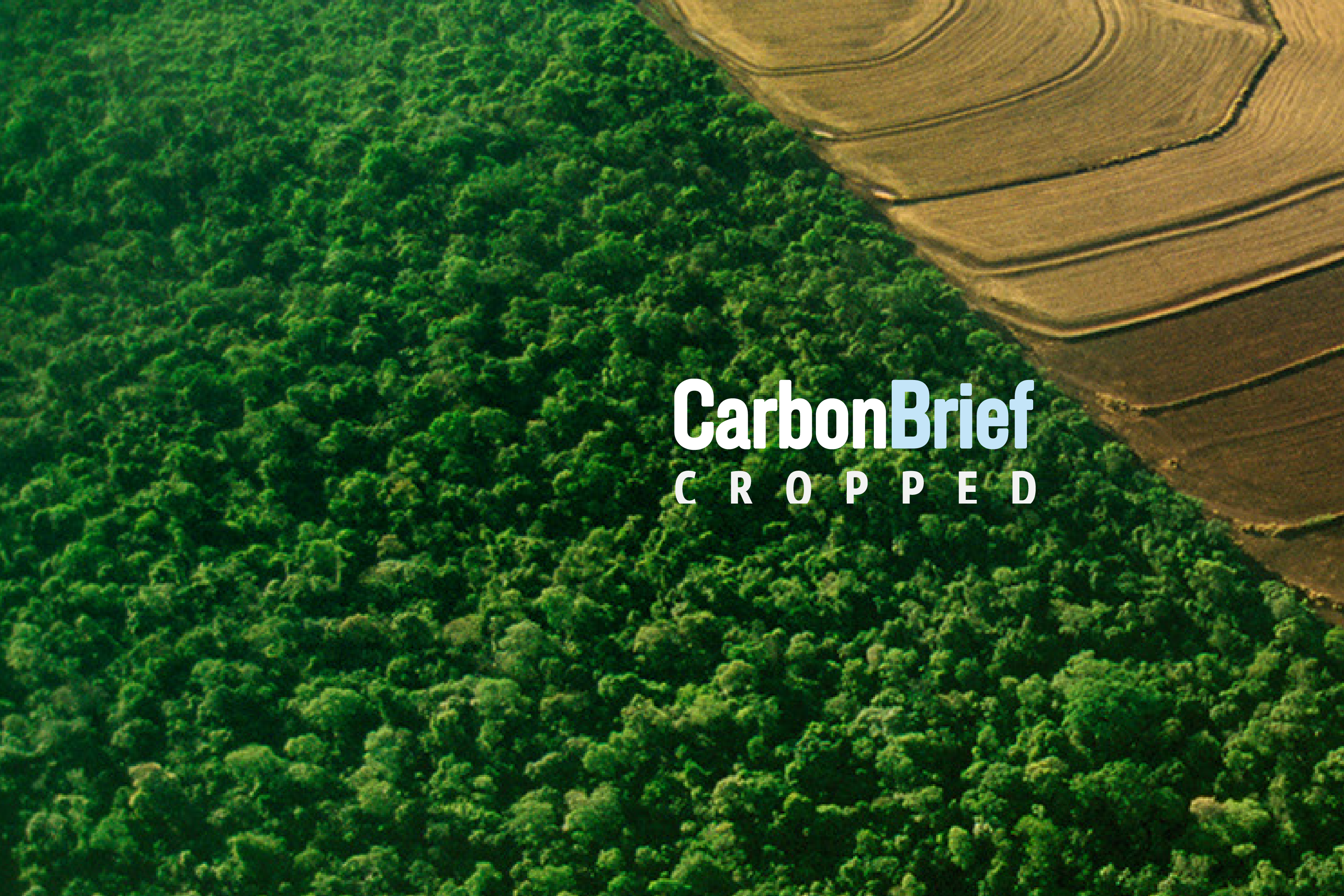This horizontally aligned rectangular aerial image provides a striking contrast between two distinct types of landscape. The entire left side is dominated by dense, lush green trees, reminiscent of a vibrant broccoli canopy. In contrast, the right side features flat, brown land that curves upward towards the upper right corner, resembling rows of cultivated fields or dirt plots, with some areas possibly used for planting crops. Centrally across the image, the words "carbonbrief" are prominently displayed, with "carbon" in bold white letters and "brief" in a light blue bold font. Beneath this, the word "CROPPED" is written in all caps, white letters. The juxtaposition of the verdant greenery against the earthy tones of farmland, combined with the textual elements, suggests a topic related to agriculture or environmental studies.